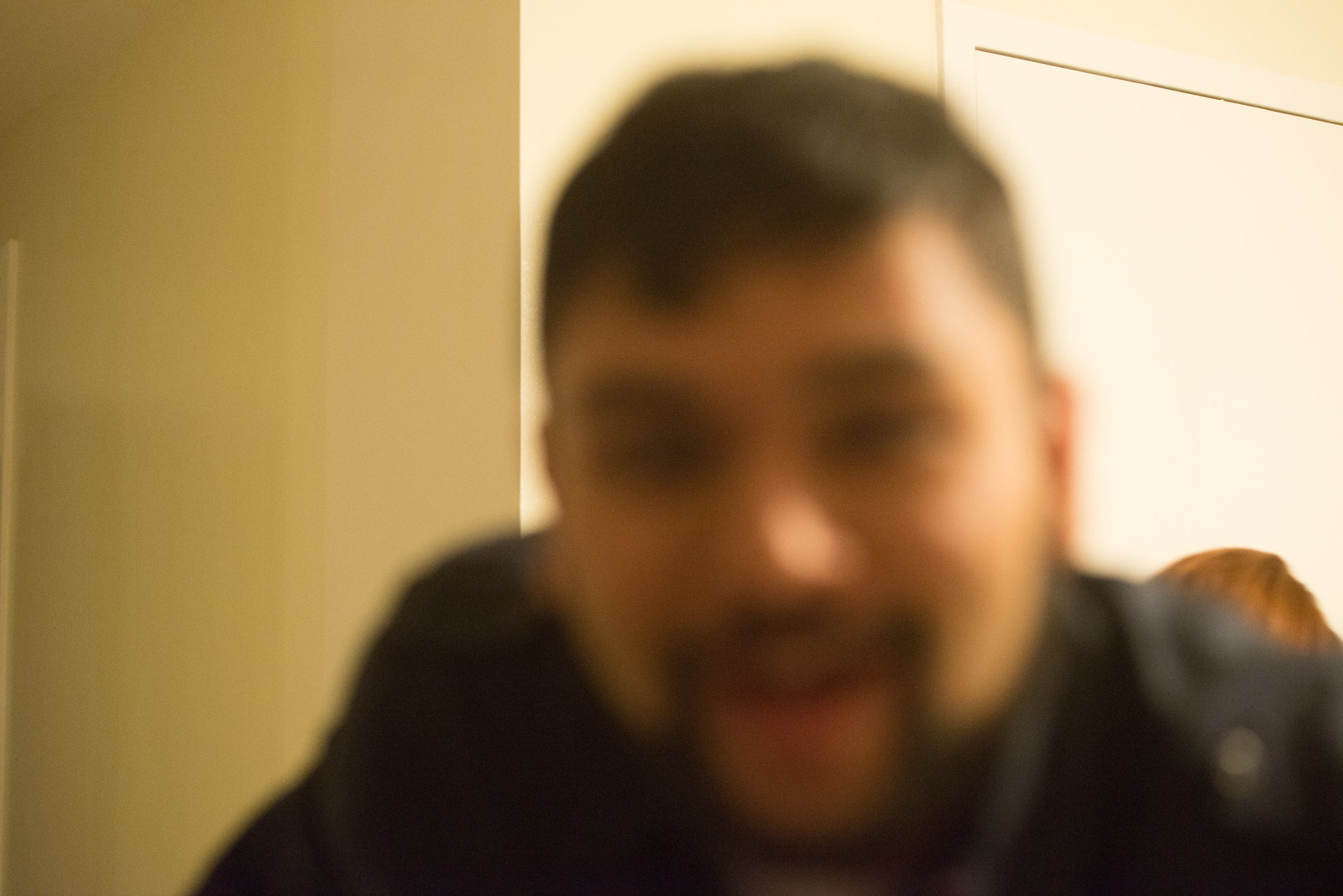In this slightly surreal and intimate indoor photograph, the close-up of a man's face occupies the entire center of the frame, though it is notably blurry and out-of-focus. His pleasant smile is discernible despite the lack of sharpness, and he sports a mustache that extends down the sides of his lips. His face has a rugged charm, with an unshaven look on his cheeks and a modest beard tracing the very bottom of his chin. The background contrasts sharply with his visage; the walls are crisp and in focus, grounding the scene in a clear setting. A light source from the right side gently illuminates his face, creating a subtle gradient of light and shadow. His hair is short and cropped, and he is dressed in a black button-down shirt, adding to his casual, approachable appearance. The juxtaposition of the blurred foreground and the sharp background evokes a sense of depth and context to the photograph.